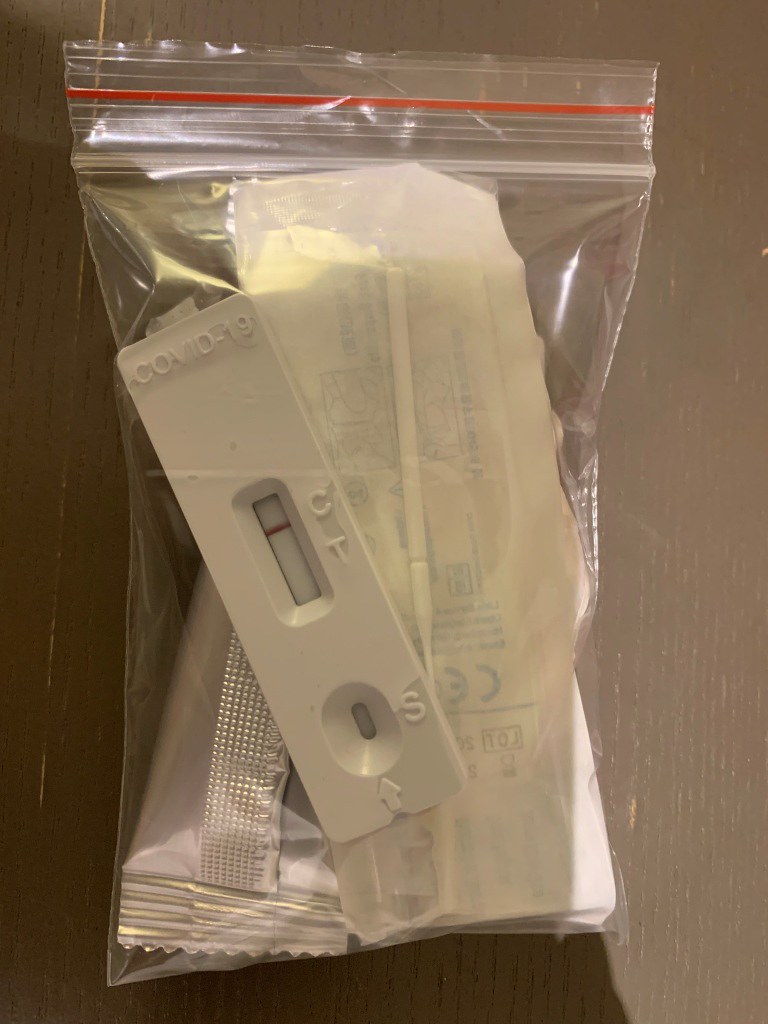In the image, we observe a desk with a rich brown wood finish. On the desk rests a small, clear plastic bag featuring a white zip closure and a distinctive red line above the zipper. Inside the bag is a white plastic COVID-19 test kit. The kit displays a single red line next to the letter "C" on the embedded test strip, indicating a negative result, as no line appears next to the letter "T." The top of the test kit prominently reads "COVID-19." At the bottom, there is an indented circle labeled with the letter "S," adjacent to an engraved arrow pointing to the sample collection hole. Additionally, the bag contains a nasal swab, enclosed within a piece of white paper, intended for sample collection. There is also an unidentifiable item sealed in a plastic wrapper accompanying the test kit.